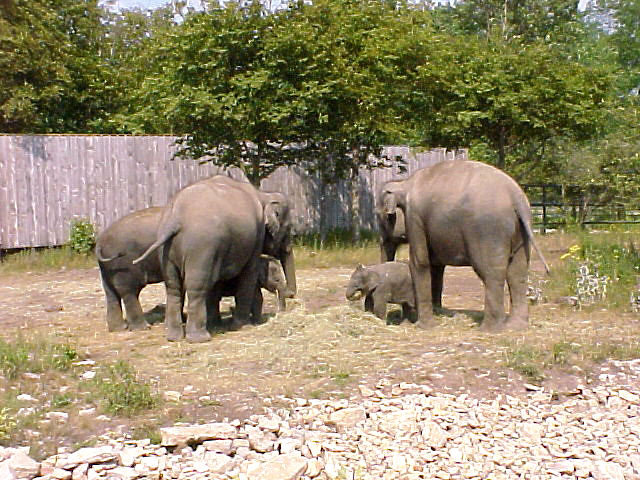The picture shows a group of four elephants, consisting of two adults, one medium-sized adolescent, and a baby, situated in a zoo enclosure. Despite the slight blurriness of the image, the elephants can be seen eating grass or hay from the ground. They are positioned such that the baby elephants are in the center, surrounded protectively by the larger adults. The enclosure features a wooden fence along the back and a metal pipe fence on the right-hand side. Surrounding the elephants are trees with green leaves, patches of scattered grass, stone paddles in the foreground, and some flowers on the left. The elephants are Asian, distinguishable by their head shape and lack of tusks and large ears.